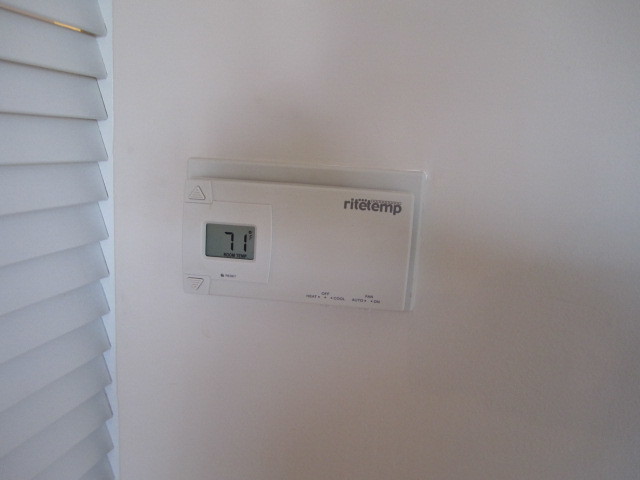This is a detailed caption for the described photograph:

In this horizontal rectangular photograph, a white background features some shadowing towards the upper portion and in the lower left corner. Positioned slightly left of center is a white rectangular thermostat. In the upper right corner of the thermostat, grey text spells out "rite temp" in all lowercase letters, with "rite" spelled "R-I-T-E" and "temp" as "T-E-M-P," forming one word. Near the bottom right of the thermostat, there's some small, unreadable text. On the left side of the device, there is a square section containing a digital screen that displays the temperature as "71°F," with the Fahrenheit symbol ("F") appearing in the upper right corner of the screen. Adjacent to the thermostat, to the left, is a wall characterized by horizontal, rectangular white planks, reminiscent of exterior siding. The planks are tiered, adding texture to the otherwise monochromatic scene. The shades of white between the thermostat and the planked wall are slightly different, providing a subtle contrast.